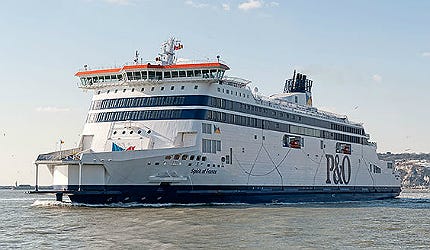The photograph, taken outdoors during daytime, captures a calm scene under a gray and blue sky with minor clouds. The rectangular image, roughly two and a half inches wide by one and a half inches tall, features a smaller, older cruise ship prominently in the frame. The lower half-inch of the picture depicts calm, grayish-brown water. Dominating the scene, slightly towards the left and foreground, the cruise ship is mostly white with a dark gray bottom. It has navy blue and dark blue paint stripes accentuating at least two rows of large windows or balconies. The captain's area features a striking orange roof, and an orange smoke stack is visible. In bold black typography, "P&O" is printed along the side. Situated in a port or coastal area, the background to the right shows a city perched on a hill, with some buildings and trees faintly discernible due to the image's low resolution.